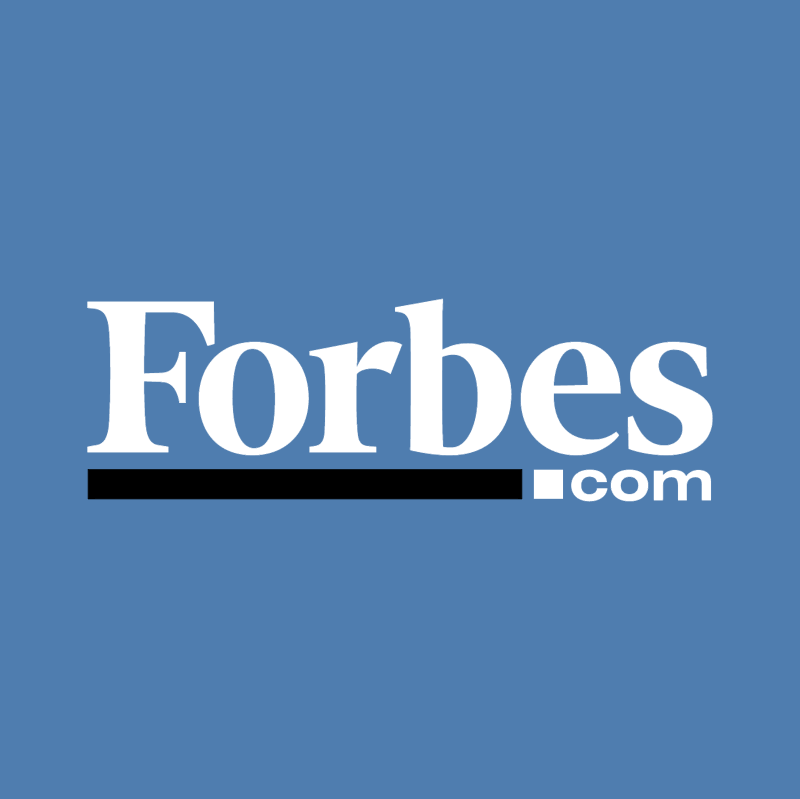The image is a rectangle with a solid light blue background, slightly taller than it is wide. In the center, large white text spells "Forbes," with the "F" capitalized and the remaining letters in lowercase. A black horizontal rectangle underlines the "F-O-R-B" of "Forbes." Directly below the "E-S" of "Forbes," in smaller white text, is "com," which makes the entire text read as "Forbes.com." The image is geometrically simple and visually straightforward, with uniform colors and no shading. The overall design is clean, minimalistic, and easy to comprehend.